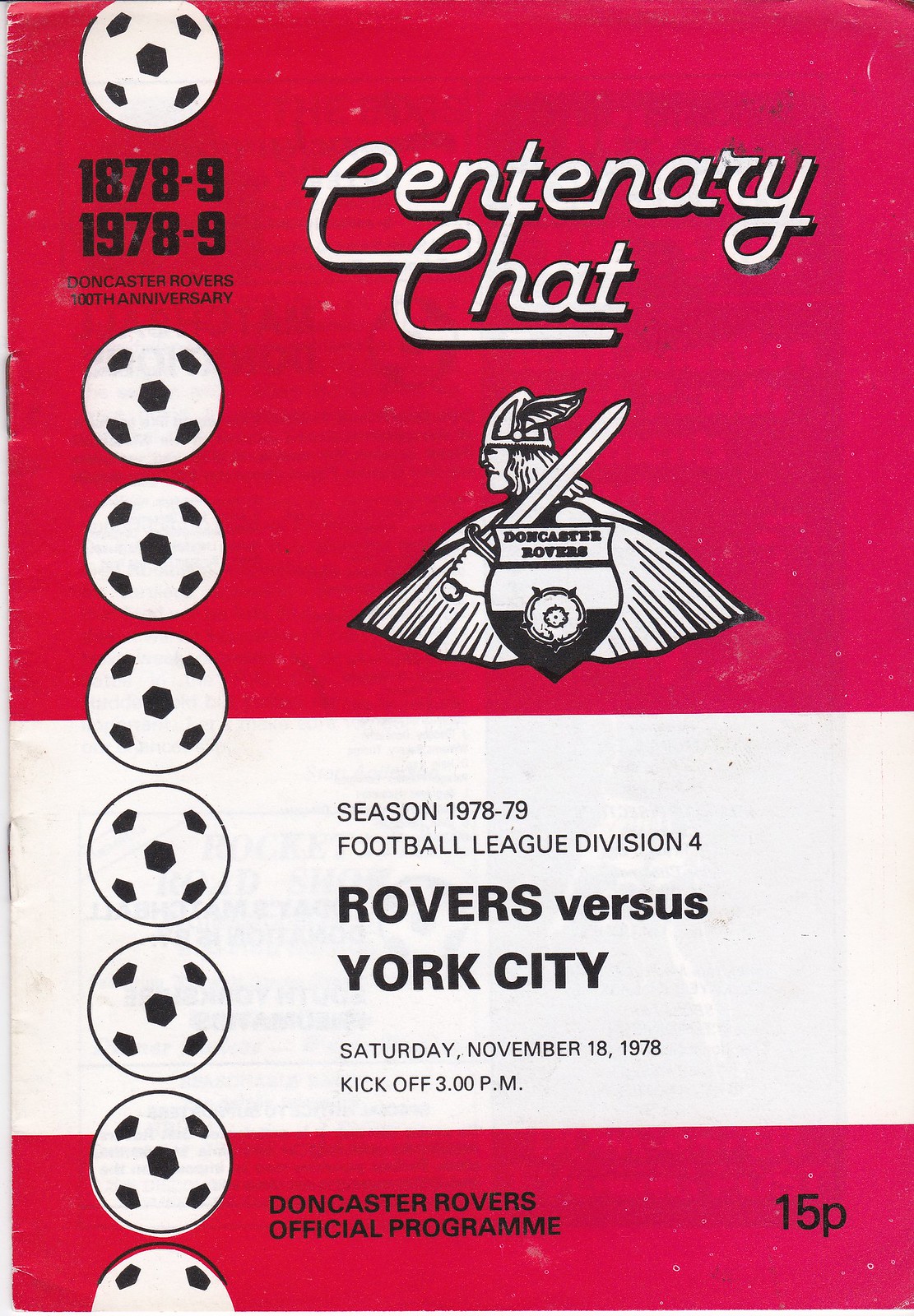The image depicts the cover of a soccer game program, characterized by a distinct red and white striped background. The design is segmented into three parts: an upper red section, a central white banner, and a lower red banner. At the top, the title "Centenary Chat" is prominently displayed on the red background. Below this, a Viking-like figure is illustrated, complete with a helmet, cape, and sword, holding a shield that bears the name "Doncaster Rovers." To the left of the Viking figure, soccer balls are vertically stacked, featuring the years "1878-9" and "1978-9," alongside the phrase "Doncaster Rovers 100th Anniversary." 

In the center white section of the program, the text announces: 
"Season 1978-79
Football League Division 4
Rovers vs York City
Saturday, November 18, 1978
Kick-off, 3pm."

Finally, the bottom red part of the cover states "Doncaster Rovers Official Program" with a notation of the cost, "15p," placed on the right-hand side.